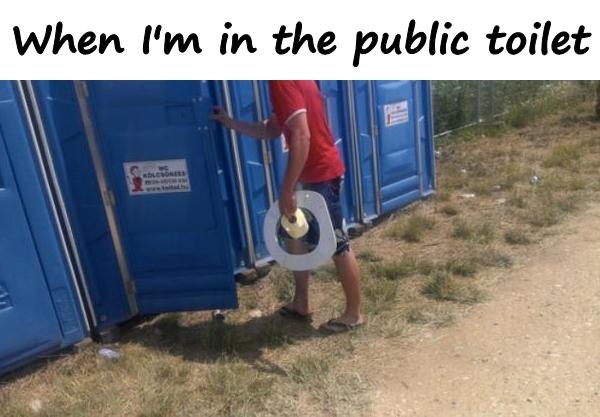The photograph captures an outdoor scene featuring a dirt road pathway with sparse, random patches of green grass. Four blue port-a-potties are aligned diagonally from the bottom left to the top right of the image. A young man, seen from the shoulders down, is captured in the act of opening the door of the third port-a-potty from the left. He is dressed in a red t-shirt, long blue board shorts, and brown flip-flops. In his left hand, he carries a white toilet seat and a roll of yellow toilet paper, while his right hand is engaged in opening the port-a-potty door. His right foot is positioned slightly in front of his left, indicating he is about to step inside. Above the image, the text "When I'm in the public toilet" is written in black font.